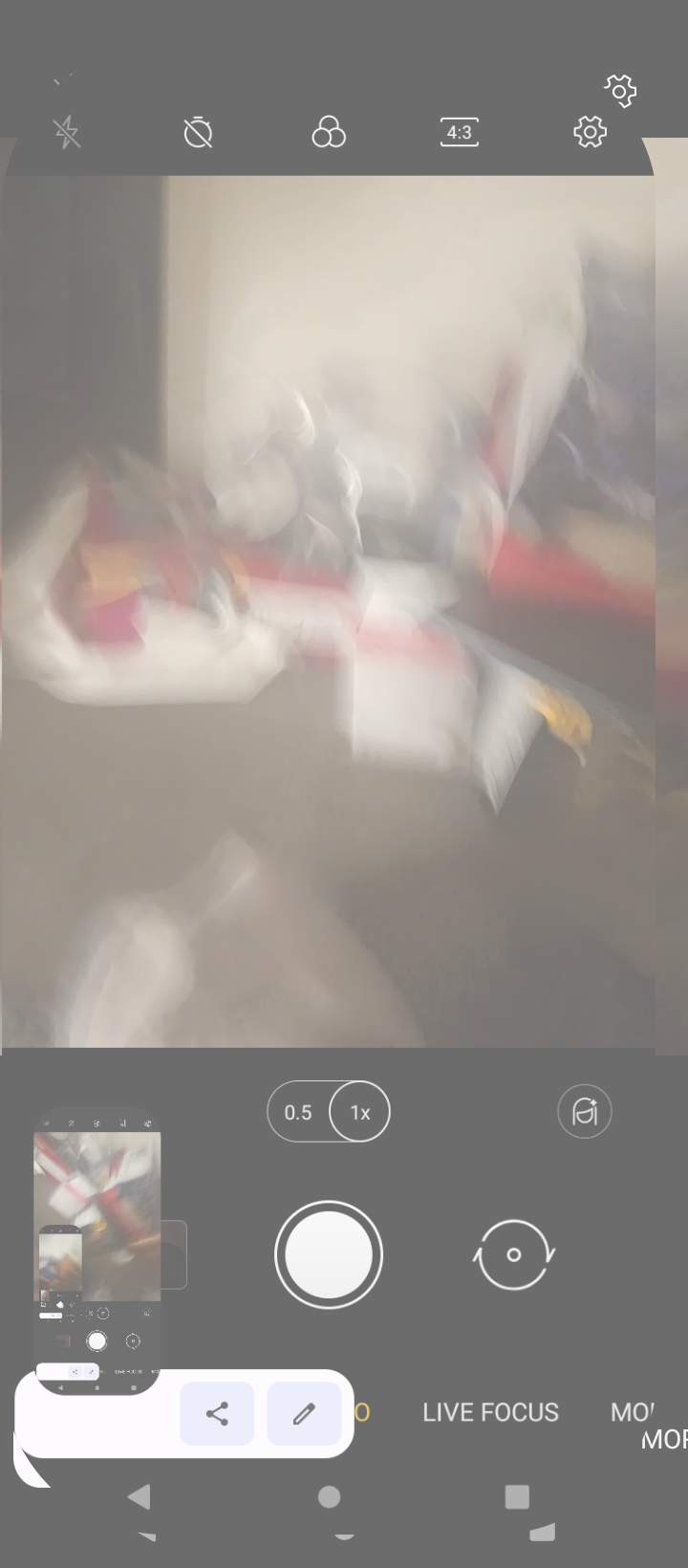A colored photograph captures a cell phone screen displaying a blurred attempt to photograph a scene, presumably featuring a collection of packages on a green floor against a white wall. The upper portion of the photo shows the phone's interface, with a black horizontal ribbon containing various camera mode icons. In the lower third, the screen is predominantly black, displaying the camera interface icons clearly. The central circular white button is prominent for taking pictures, flanked by a focus button labeled "0.5" and a zoom indicator marked "1X". The term "live focus" appears in capital letters, slightly cut off toward the right. Although the photograph is too blurry to distinguish details clearly, the colors red, yellow, white, and black are noticeable, suggesting a possible Christmas scene with gifts. The photograph also shows additional icons such as the share and edit symbols, against a dark brown, almost black background, with white illuminated icons indicating various functions of the camera mode.